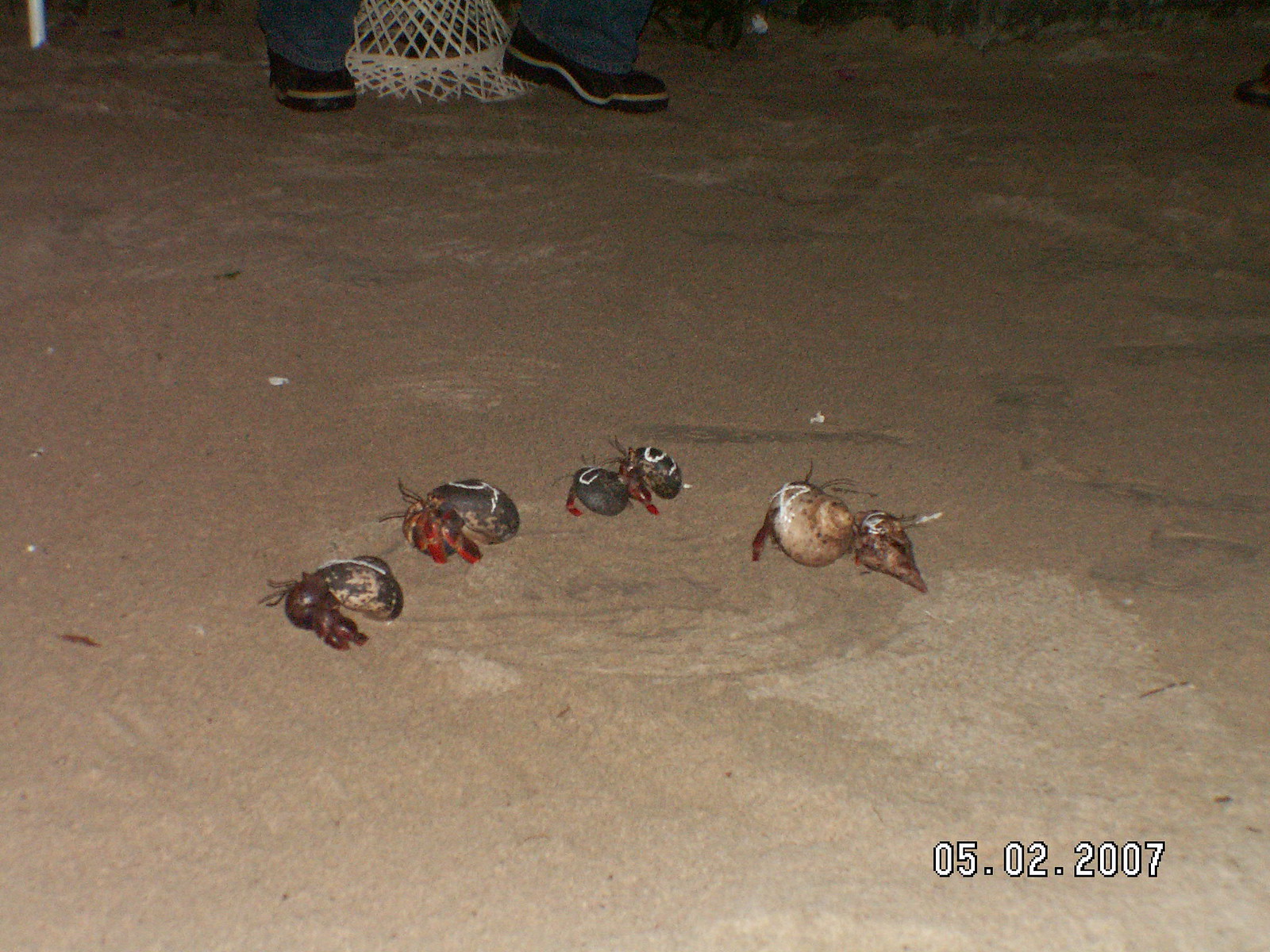The color photograph, dated 05.02.2007 in white text with a black outline in the bottom right corner, showcases a beach scene at nighttime illuminated by a flash. In the center of the photograph, an arc formation of various sea creatures, possibly crabs or snails, is slightly out of focus. These creatures, set against a sandy or rocky surface, exhibit an assortment of sizes, colors, and orientations—some appear to be moving in different directions. Notably, one of the animals features a grey shell with white circles, another has a pale beige shell with white markings, while others are red or brown with distinct patterns, such as red legs or prominent circles on their shells. The background reveals a much darker area compared to the illuminated foreground, suggesting a nighttime shot. Additionally, at the top of the image, partially visible are a pair of feet in black and white shoes, possibly boots, standing next to a white mesh bag. The contrast in lighting heightens the nocturnal atmosphere of this compelling beach scene.